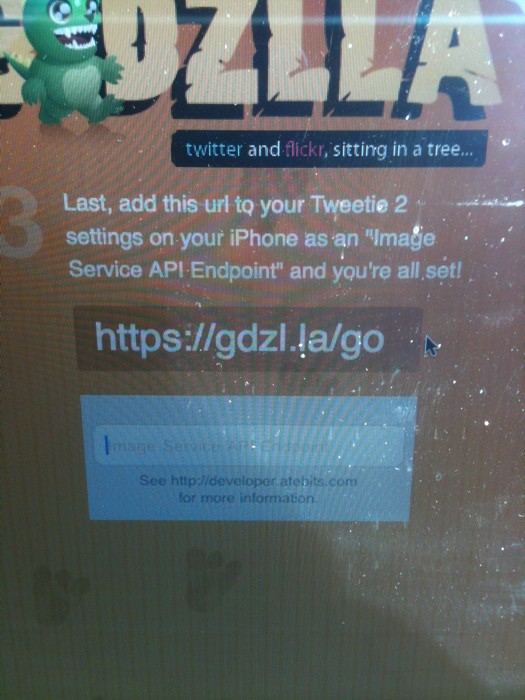The image appears to be a photograph of a computer monitor displaying a website, featuring visible dust, grime, and a shadow over the lower left half. Dominating the layout, the text "Godzilla" in uppercase yellow letters spans the top, accompanied by an illustration of a small green Godzilla-like cartoon character. Below it, a black rectangle bears the playful phrase "Twitter and Flickr sitting in a tree," with "Twitter" rendered in light blue and "Flickr" in pink. The instruction "Last, add this URL to your Tweety2 settings on your iPhone as an image service API endpoint and you're all set" follows, complemented by a URL. Beneath the URL, a white text input field labeled "image service API endpoint" is present, with no text being entered, set against a brown background. The URL displayed is https://gdzl.la.la.gov, and additional information could be found at another URL labeled chttp://developerbeefbits.com.